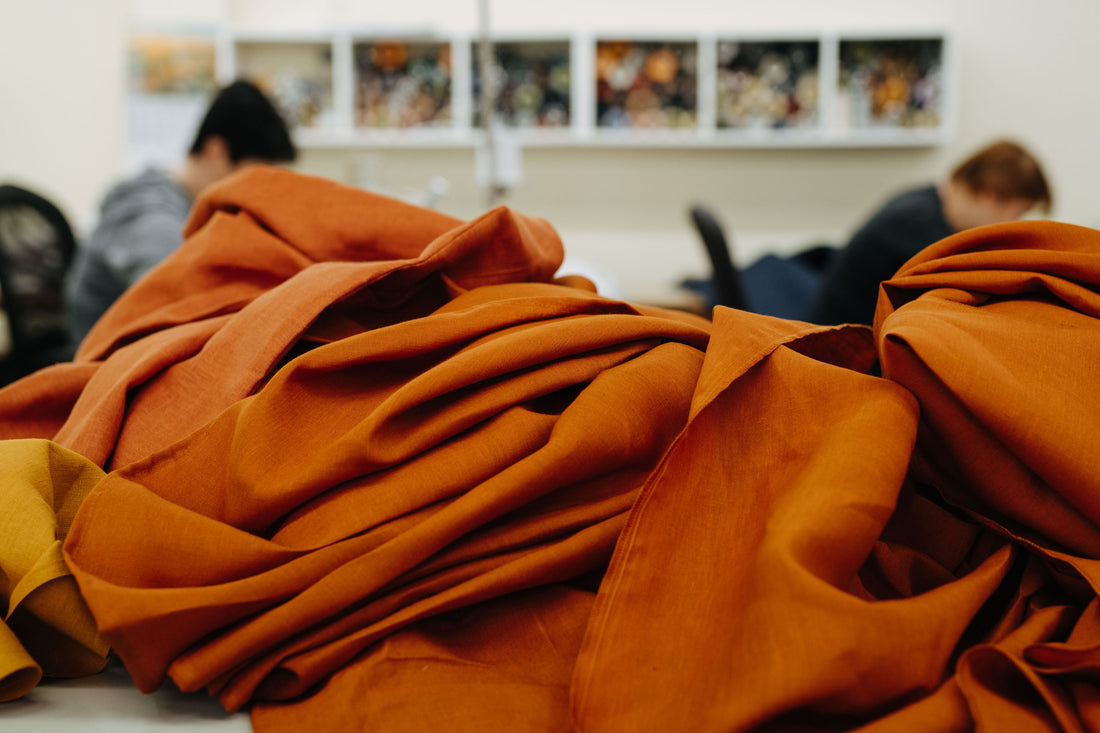In a room with a beige wall, a photograph captures a scene dominated by a large, rumpled piece of orange and yellow cloth lying prominently in the foreground. This cloth could be fabric for a sewing project or a discarded piece of clothing. In the background, slightly blurred, are two individuals seated in black office chairs. On the left, a young man in a green hoodie leans forward with his head tipped down, appearing to read something on the table in front of him. To the right, another person with brown or red hair, dressed in a dark shirt, also looks downward at their desk. Above this person, a line of seven framed images, each housed in wooden frames, protrudes from the wall, enhancing the workshop-like vibe of the setting. The background also seems to suggest a cluttered workspace, hinting at shelves or cupboards potentially holding bolts of fabric, emphasizing the creative atmosphere.